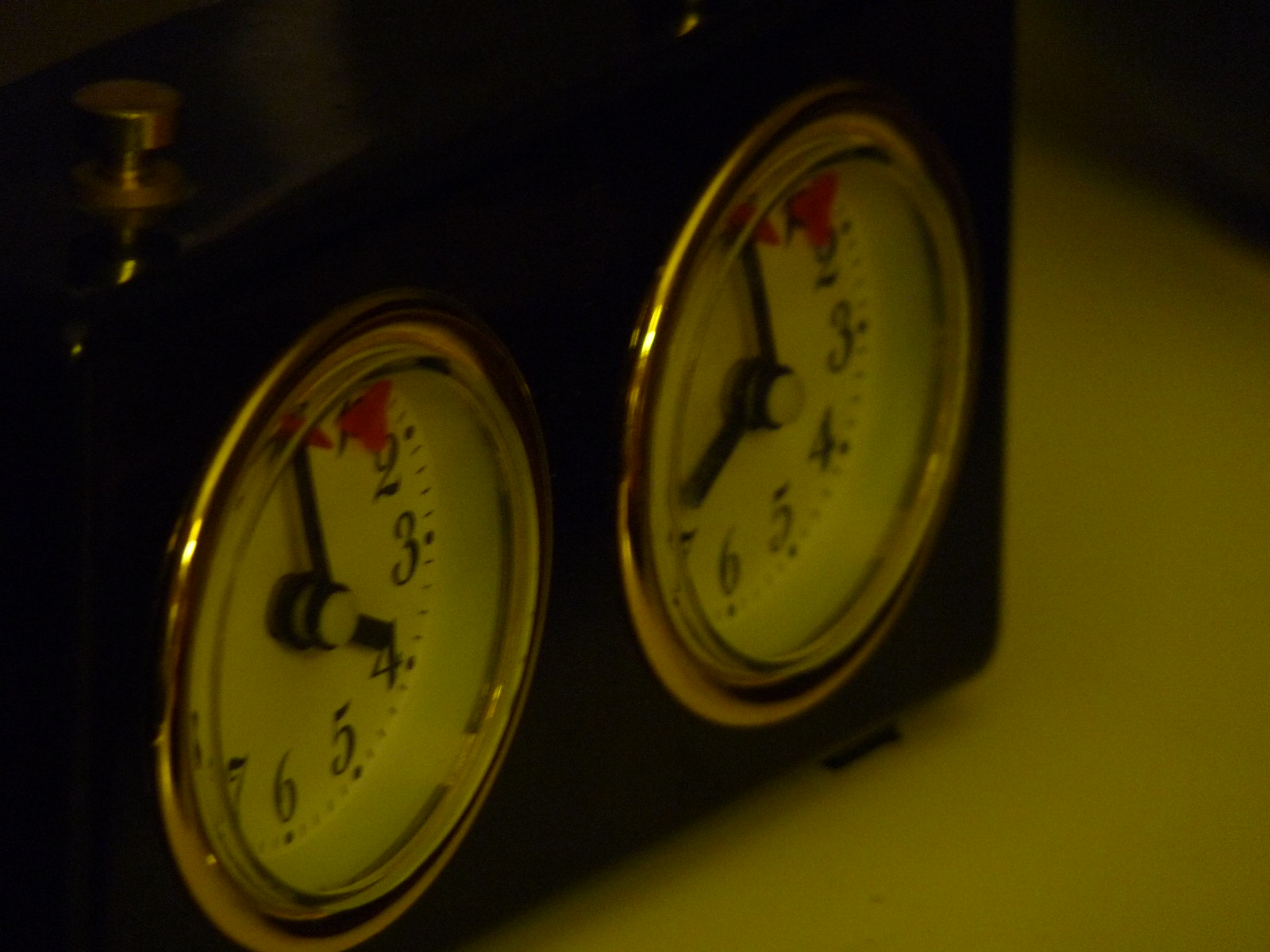This close-up image, slightly blurry and dimly lit, captures two round clock faces embedded in a dark wooden rectangular frame. Each clock face is encircled by a brass ring and features a white background with black numbers. Both clocks have black hands with a white button at the center holding them in place. The clock on the left indicates the time as four o'clock, while the clock on the right displays seven o'clock. Near the twelve and one positions on each clock, small red arrows are visible. The wooden frame housing the clocks rests on a white surface, adding contrast to the overall composition.